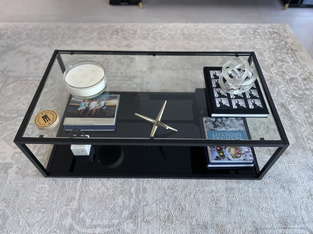This image showcases a sleek, modern glass coffee table with a black metal frame, stylishly situated on a light-colored, textured rug. The top surface of the table is carefully curated with various items. On the left side, there is a round white candle in a glass container, emanating a cozy ambiance. Adjacent to the candle is a neatly stacked pile of books, with the topmost book featuring a vibrant cover displaying an image of people. Placed atop this stack is a coaster adorned with a logo. On the right side of the table, two smaller book stacks are present. The stack closest to the center features a book with a striking black and white cover embellished with small images. The further right stack is topped with a book bearing a colorful cover and some indistinct text. The lower shelf of the table, made of a dark and glossy material, remains elegantly empty, adding to the minimalist aesthetic. The overall design exudes a modern yet minimal feel, though the apparent fragility of the glass top might be a concern regarding its durability. It is unclear if the sides of the table are also encased in glass.